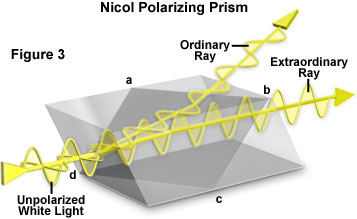The image showcases a labeled diagram on a plain white background, centered around a semi-transparent, grayish 3D prism, identified as the "Nicol Polarizing Prism" (incorrectly named as "Nicole Polarizing Prism" in one description). Despite being blurry and low in quality, the depiction is moderately detailed. The top left corner of the image includes the label “Figure 3” in black text. The prism itself has a complex structure with visible lighter and darker shades, enhancing its three-dimensional appearance.

Above the prism are two yellow, wavy arrows. The arrow starting from the bottom left, labeled “Unpolarized White Light,” strikes the prism. Upon entering, this ray splits into two distinct paths: one arrow, labeled “Ordinary Ray,” bends upwards and exits through the top of the prism, while the other, labeled “Extraordinary Ray,” continues straight and exits through the opposite side. The meticulous labeling and arrows provide a clear interpretation of the light behavior when passing through the prism.